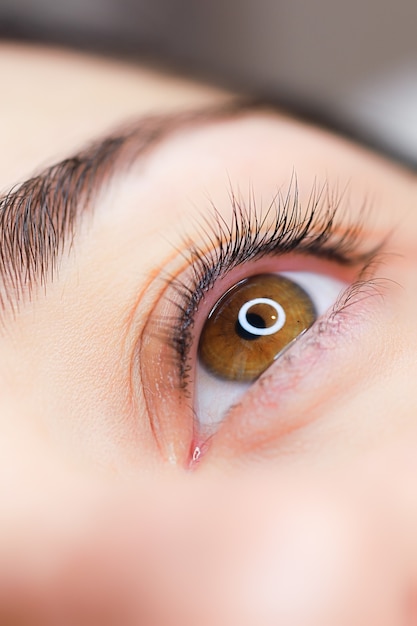In this super close-up, highly detailed image, we focus on the left eye of a young Caucasian woman. Her eye is a vivid golden-brown, sharp and clear, reflecting a circular ring light that creates a striking, bright white ring around her black pupil. Surrounding this captivating eye, her eyelashes curl upwards, thick and black on the top, yet notably sparse on the bottom, revealing bare skin underneath. Her eyebrows, sparse and thin towards the outer edge, are also black, contributing to her overall delicate appearance. The skin around her eye is pale and clear, indicating youth, as it lacks any visible makeup, wrinkles, or bags. The minimalism of the surrounding visible area focuses all attention on her eye and its immediate features, suggesting a natural beauty.